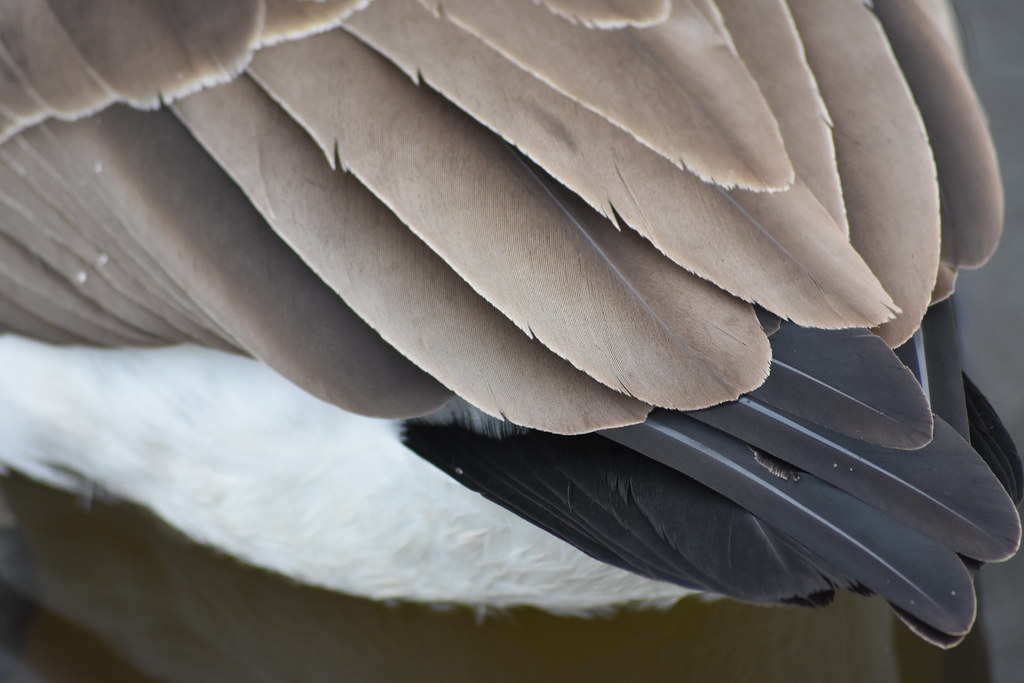This close-up image showcases the delicate tail feathers of a Canadian goose. The focus is solely on the tail, highlighting an intricate combination of colors and textures. At the very top, we see a layer of light mocha brown feathers, neatly folded and overlapping one another, creating a harmonious array. These feathers fade into darker shades towards the middle, accentuated by natural shadows. Just beneath this is a row of black feathers, each marked with a thin, white line running through their center, adding a striking contrast. The very bottom of the tail is adorned with fluffy, pure white feathers, reminiscent of soft pillow stuffing, which appear slightly out of focus. The backdrop of the image features a reflective surface that suggests the bird is perched by a lake, enhancing the serene and natural setting. No other parts of the bird are visible, making the tail the central subject of the photograph.